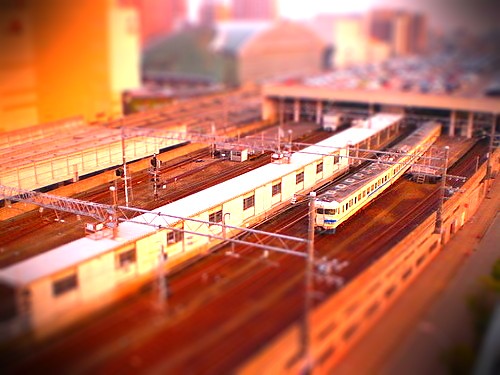The image depicts a vibrant, sepia-toned scene, likely captured at sunrise or sunset, enveloping a train yard or railway station with an ethereal glow. The central focus is a butter-yellow train with distinctive blue stripes gliding on tracks tinged with an orangey hue. The composition, enhanced by the unique angle and color palette, lends the photo a miniature, almost toy-like appearance, though it captures a real setting. Surrounding the train are various buildings, a possible parking lot, and utility poles, all contributing to the urban backdrop. These elements blur into the background, giving the scene a dreamlike, vintage ambiance, reminiscent of the 1970s. Black marks gently fade at the edges of the image, adding to the photo’s nostalgic and intriguing aesthetic. All in all, it's a captivating blend of vivid colors and blurred peripheries, framing an old-world railway scene brought to life.